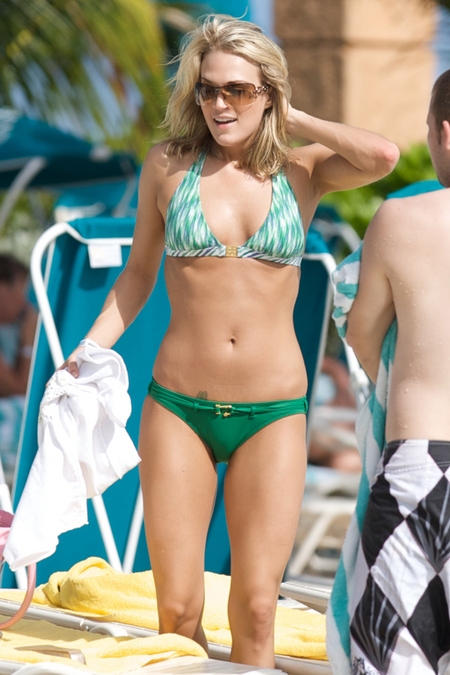The photograph appears to be a candid shot of a woman who closely resembles Reese Witherspoon on a beach, wearing a mismatched green and white bikini. Her blonde hair falls to shoulder length, and she is wearing sunglasses. The bikini top is a light green with white, while the bottom is solid green and features a small green belt with a gold buckle. A subtle tattoo is visible just above her bikini line on the left side. She is holding a white towel in her right hand and adjusting her hair with her left. In the background, a large column reminiscent of the Arc de Triomphe and a palm tree add to the beach resort setting. A man, holding a towel, stands to the right of her, possibly looking at her, while numerous beach chairs, umbrellas, and a glimpse of a teenage boy are also visible.